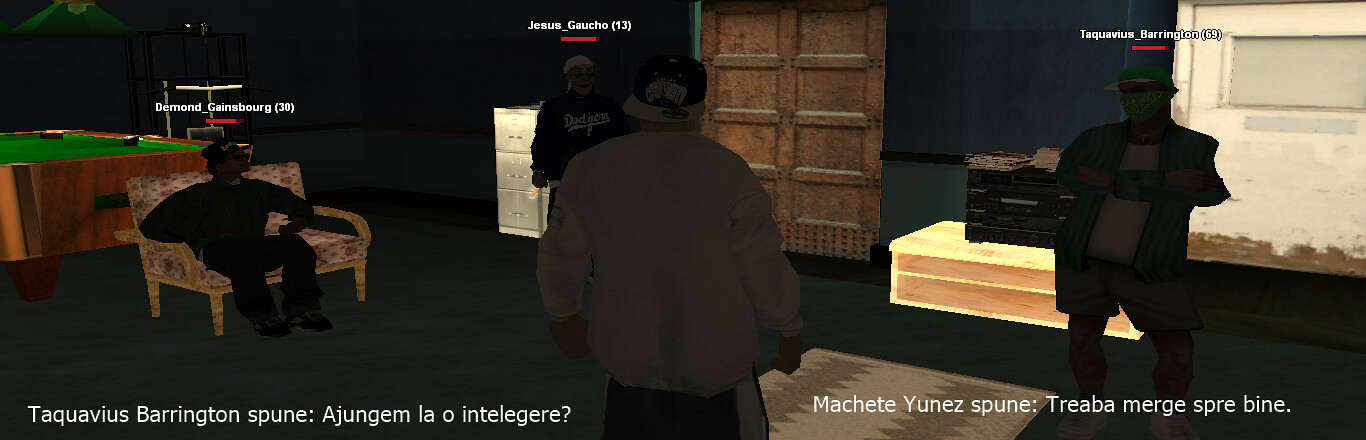### Descriptive Caption

In this frame captured from a multiplayer video game, we see the back of the main player, prominently positioned in the center of the screen. They are dressed in a large white jacket paired with what resembles basketball shorts or long track jeans. Surrounding the main player are three other avatars, each engaged in varying poses and interactions. 

On the left-hand side, a player identified as Demond_Gainsburg is seated on either a table or a seat. Directly ahead facing the central character stands Jesus Gacho, while to the right, another player named Tequavious Barrington also stands and faces the main character. The setting appears to be indoors, characterized by a large wooden door centrally located in the background and another white door to the right.

Additional details of the environment include a filing cabinet on the left, a pool table positioned further to the left, dark green carpeting covering the floor, and a white runner rug placed towards the center. On the right side, shelving units adorned with various items add to the intricate detailing of the room's furnishings.